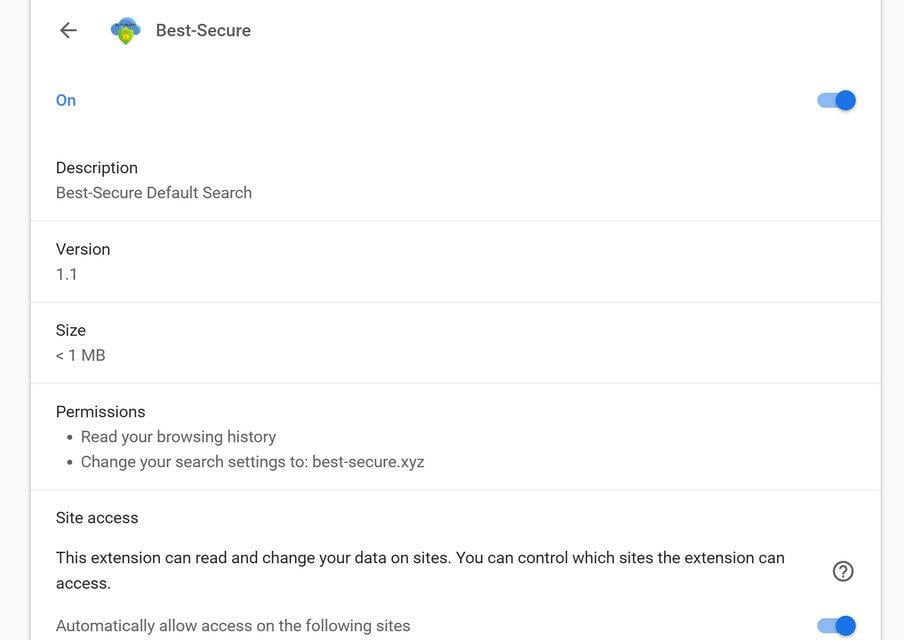**Detailed Caption:**

The image depicts a computer screen displaying the settings page of a browser extension called "Best Secure." The interface features an all-white background with a text-based layout. At the top of the screen, the title "Best Secure" is visible, accompanied by a small green and blue logo. A black arrow pointing left indicates the option to go back to the previous page.

In the header section, the text "On" is written in blue letters, positioned centrally, with a blue toggle switch on the far right, indicating that the extension is currently enabled. Below this, a section labeled "Description" is seen, alongside non-bold text stating "Best Secure Default Search," followed by a horizontal gray line.

Further down, the "Version" section is in bold with "1.1" noted underneath, separated by another gray line from the "Size" section, which is also bold and mentions "1 megabyte" with a caret symbol. This is followed by another gray line. 

The "Permissions" section lists two bullet points: "Read Your Browsing History" and "Change Your Search Settings to bestsecure.xyz." These permissions are highlighted in bold at the beginning.

Another horizontal gray line appears, leading to a side access cautionary note: "This extension can read and change data on-site, so you can control which sites the extension can access." To the right of this note, there is a circle icon with a question mark.

At the bottom of the screen, in gray text, it states "Automatically Allow Access on the following sites," accompanied by another blue toggle switch that is also in the "On" position, located on the far right of the text.